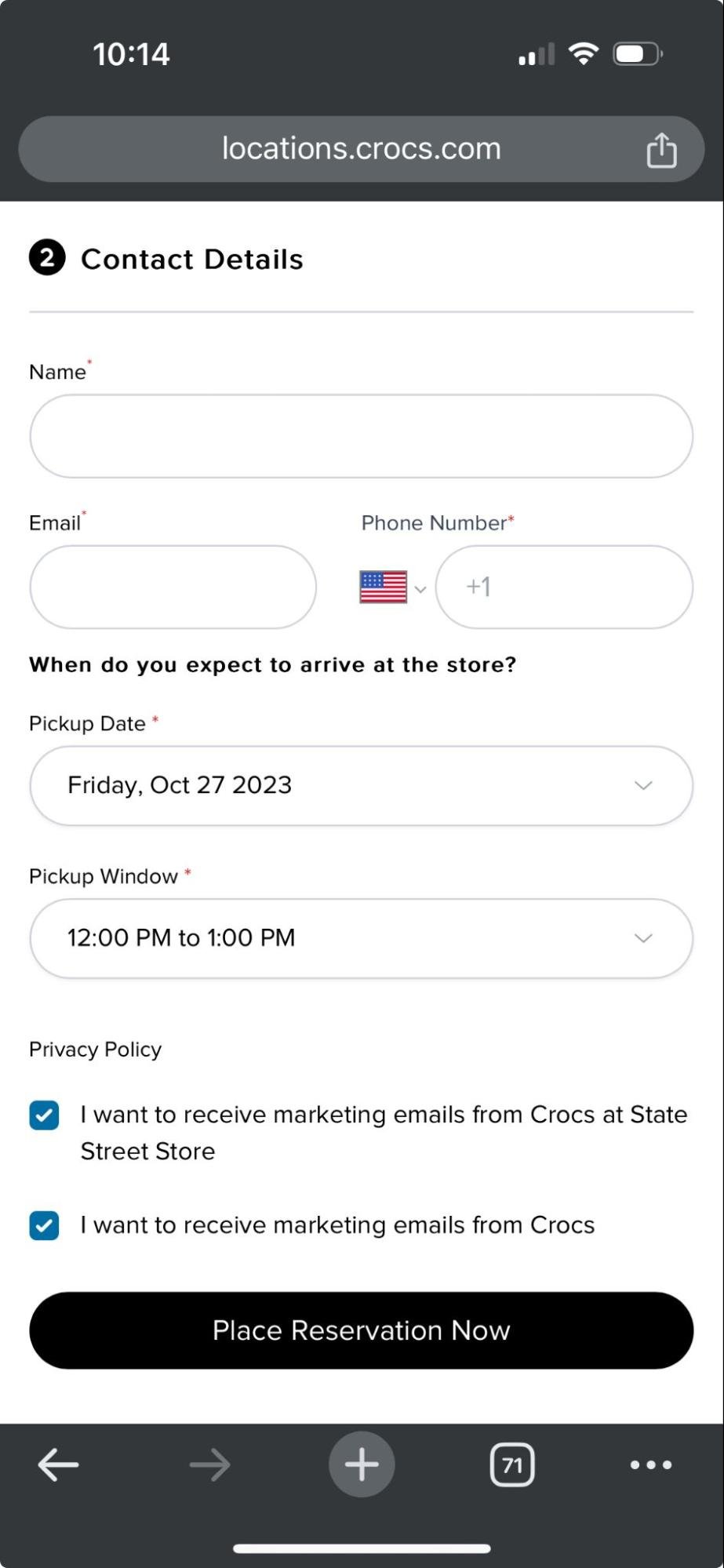Screenshot of the Crocs Website Reservation Form on a Mobile Device

At the top of the mobile screenshot, the status bar displays the time as 10:14 AM in the left corner, with Wi-Fi signal strength, cellular signal strength, and battery life indicators in the right corner. Below this, the address bar shows the URL: locations.crocs.com.

The focal point of the image is a reservation form titled "Contact Details," highlighted by a small black circle with the number two inside it. The form consists of several input fields. The first field prompts the user to enter their "Name." Following this, the next row includes fields for "Email" and "Phone Number," with a country selection dropdown showing the US flag, indicating the selection of the United States.

Further down, the form asks, "When do you expect to arrive at the store?" with fields for selecting a "Pickup Date" and a "Pickup Window." The current selections are Friday, October 27th, 2023, from 12 PM to 1 PM.

At the bottom of the form are privacy policy statements, each with a checkbox. The first statement reads, "I want to receive marketing emails from Crocs at State Street Store," and the second says, "I want to receive marketing emails from Crocs." Both checkboxes are ticked.

Finally, a prominent block button at the bottom of the form is labeled "Place Reservation Now," inviting the user to finalize their reservation.